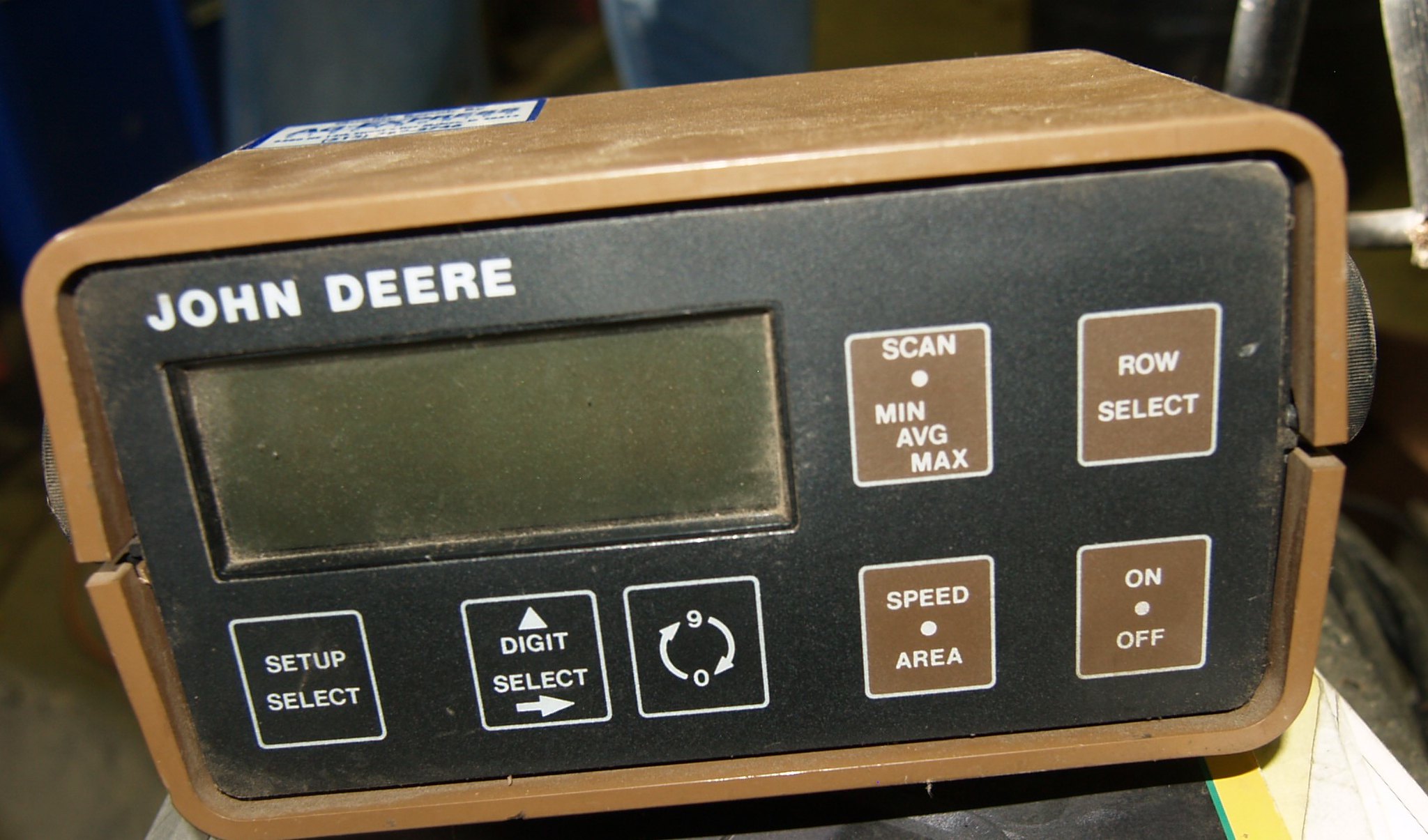This image features an old and seemingly dirty John Deere piece of equipment encased in a brown, wooden or plastic housing. The device has a rectangular shape with a black front face, prominently displaying the "John Deere" name in white uppercase letters in the upper left corner. The front face contains an inactive, blank digital screen with an olive green tint. Directly beneath the screen are three black square buttons outlined and labeled in white: "Setup Select" on the left, "Digit Select" in the middle with upward and rightward arrows, and a button featuring rotating arrows pointing from nine to zero and zero to nine. On the right side of these buttons are several brown square buttons bordered and labeled in white, arranged in a grid. The top row includes "Scan," a filled dot, "Min," "Ave," "Max"; directly below are "Row Select," "Speed," "Area," and in the lower right corner, "On" and "Off," separated by a white filled dot. There are knobs on each side of the device's casing, contributing to its utilitarian design. Additionally, a blue and white sticker appears partially visible on the top of the device, and it's placed on a black, yellow, and white surface, with indiscernible objects and small metal rods in the background.